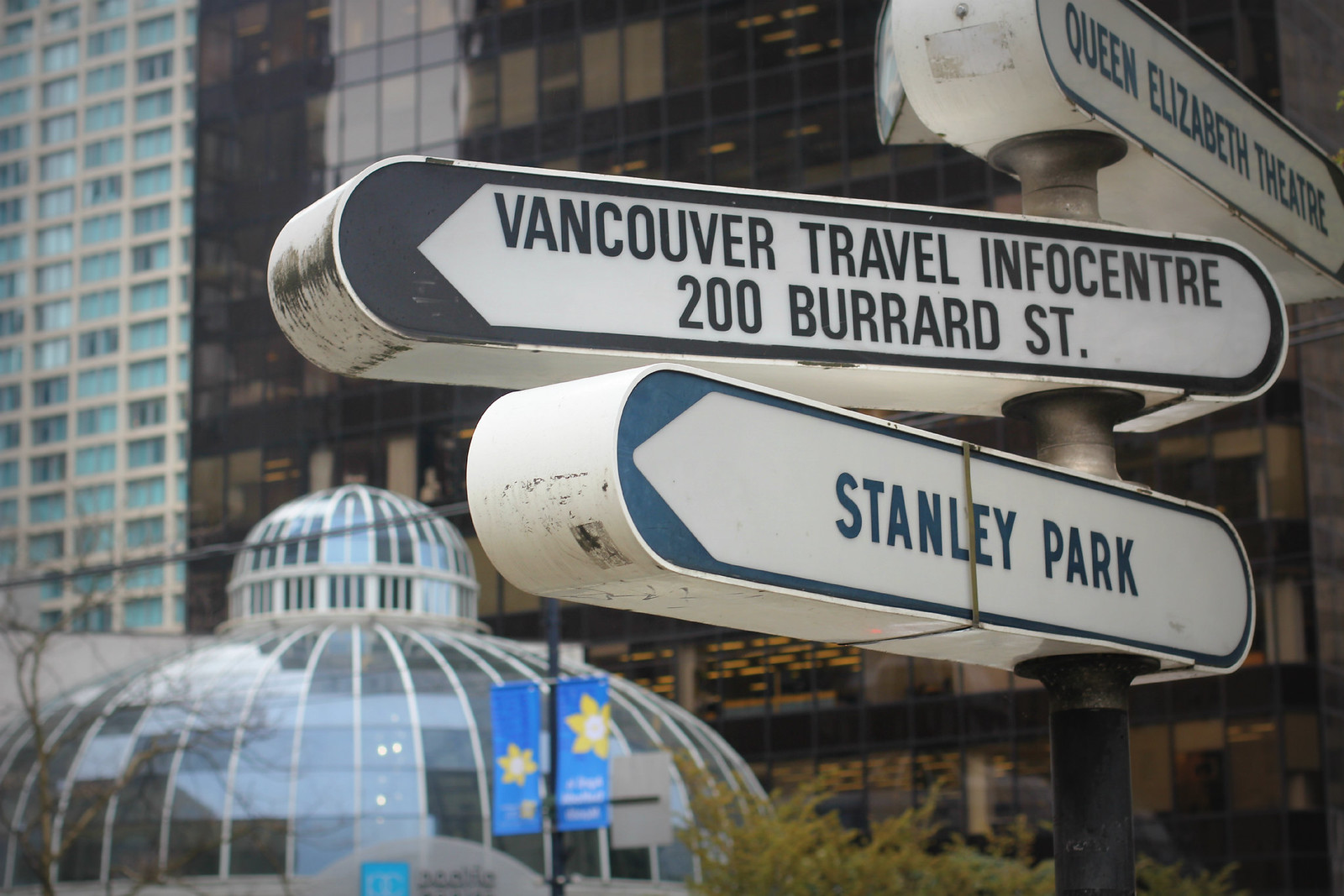In this horizontally aligned rectangular image of a city scene, the background reveals towering high-rise buildings that loom large, their tops cropped by the picture’s frame. The far left of these buildings features a brownstone facade with numerous windows, likely a hotel. Adjacent to it is a modern high-rise, brown and black, with lively interior lights visible. Down below on the lower left, there's a smaller gray building capped with a domed roof, punctuated by black windows.

In the foreground on the right side of the image, three prominent, oval-shaped, white street signs are attached to a black metal pole. The uppermost sign, angled away from the viewer, reads "Queen Elizabeth Theater" in dark blue letters. The middle sign directs left and offers practical information, saying "Vancouver Travel Info Center, 200 Burrard Street" in black text. The bottom sign, pointing generally to the right, indicates "Stanley Park," again in dark blue letters. These signs, while functional, also add a touch of character to the urban scene, guiding passersby to key locations in what seems to be a bustling part of the city.